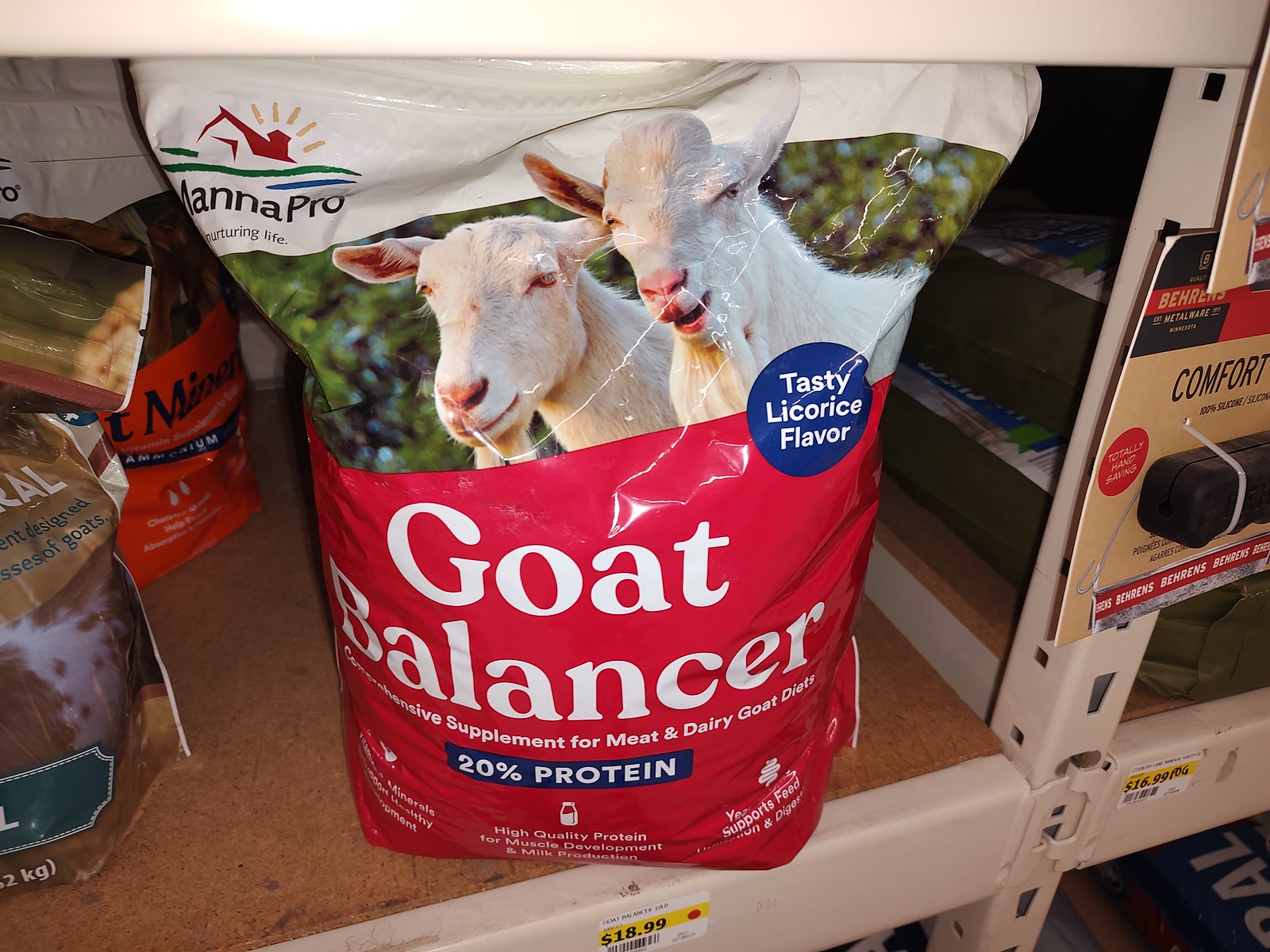The photograph captures a product displayed on a powder-coated white metal shelf in a store. The top portion of the image reveals the underside of the shelf above. The focal point is a product in the center, packaged in a mostly red plastic bag with white accents. The top of the bag features a white strip with the text "MannaPro Nurturing Life." Below this, a photograph depicts two goats standing side by side against a leafy background. Adjacent to this image is a round, blue badge indicating the product's "Tasty Licorice Flavor." The main text on the bag reads "Goat Balancer" in white letters, followed by the description "Comprehensive Supplement for Meat and Dairy Goat Diets, 20% protein."